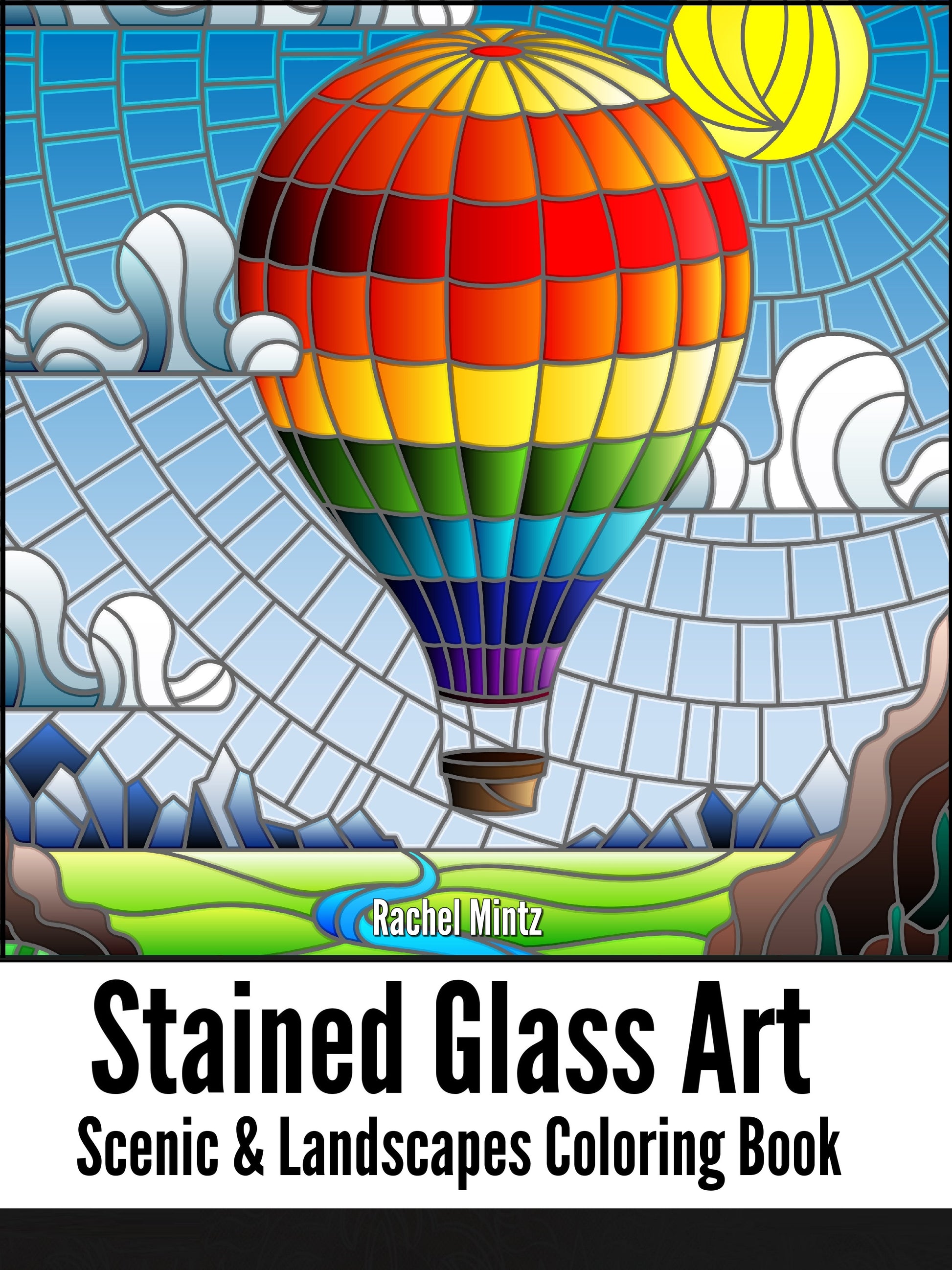The front cover of the book titled "Stained Glass Art: Scenic and Landscapes Coloring Book" by Rachel Mintz features a vibrant stained glass-style image. The artwork is intricately divided into small square and rectangular pieces and showcases a rainbow-colored hot air balloon soaring against a sky of varying blue shades, dotted with clouds. In the upper right corner, the sun shines brightly. Below, the landscape is adorned with brown and blue mountains, lush green grass, a flowing blue river, and some rocks along the corners, creating a picturesque scenery. The header text of the book, placed above the image, is in black and white, adding a classic touch to the otherwise colorful and dynamic illustration.